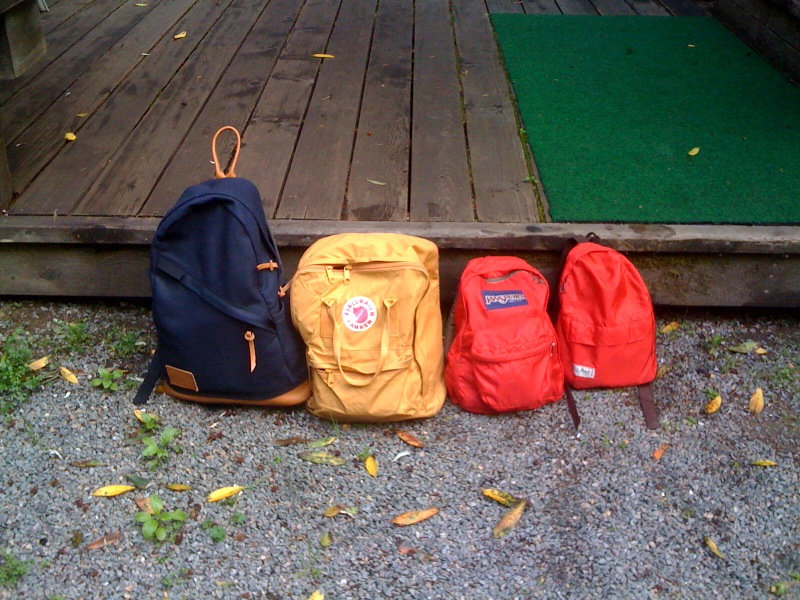The image depicts an outdoor scene with four distinct backpacks arranged in a line, positioned on a gray gravel surface scattered with leaves and plants. The backpacks, which vary in size from largest to smallest, occupy the middle third of the image, spanning from roughly 20% to 80% across the width. They are set against a darker brown wooden deck that has a few leaves scattered on it, and rises about an inch above the ground. 

Starting from the left, the first and tallest backpack is a dark blue with light brown leather-like straps and zippers, featuring a handle at the top. The second backpack is a medium yellow, decorated with a small white circle and a red emblem. The third and fourth backpacks are both a bright red, with the third one bearing the recognizable Jansport brand name on a blue square. Adjacent to the deck on the right is a patch of green astroturf, a striking contrast to the natural elements. To the left side of the deck, there seems to be an unspecified object placed upon it, adding to the rustic atmosphere of the setting.